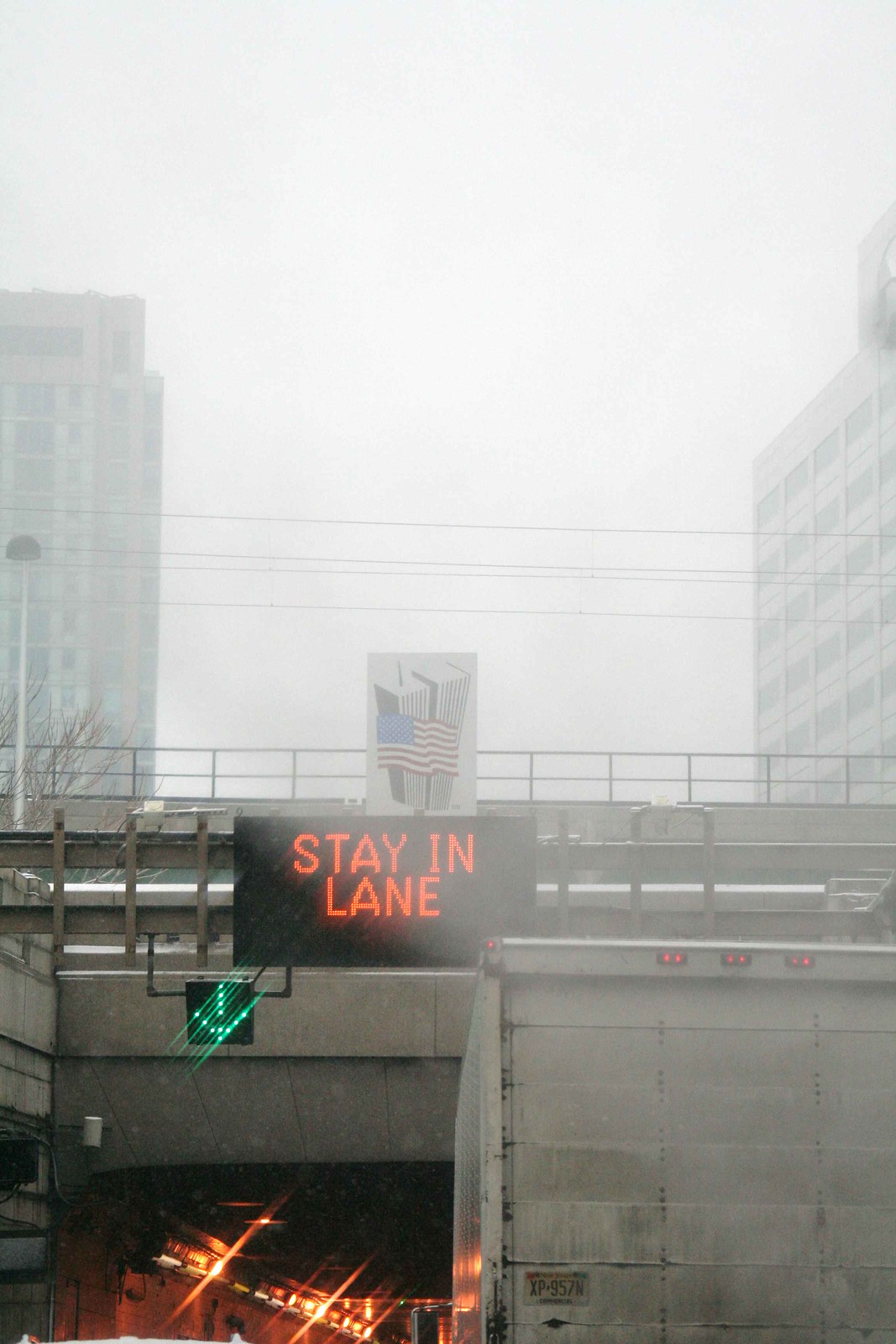This photograph, likely taken in an American city from inside a car, captures a cloudy, overcast day. The image presents a view of an underpass or tunnel, which appears to be a bridge carrying either trams or vehicles, though none are visible on it. Tall, skyscraper-like buildings flank both sides of the scene in the distance. Overhead power lines run parallel to the bridge. 

The road ahead features a black sign with bright orange letters reading “STAY IN LANE,” a directive aimed at maintaining traffic order. Below this, a lit green arrow points towards the entrance of the tunnel, which is illuminated by lights on its ceiling and sidewalls. The sky, occupying the top third of the portrait-oriented photo, is a dull white-grey, indicative of heavy cloud cover. 

In the bottom right-hand corner of the image, the back of a truck with a large container is partially visible, emphasizing the everyday rush of city traffic. Above the entrance of the tunnel is a poignant memorial image of the Twin Towers with an American flag, adding a touch of solemn patriotism to the urban scene.